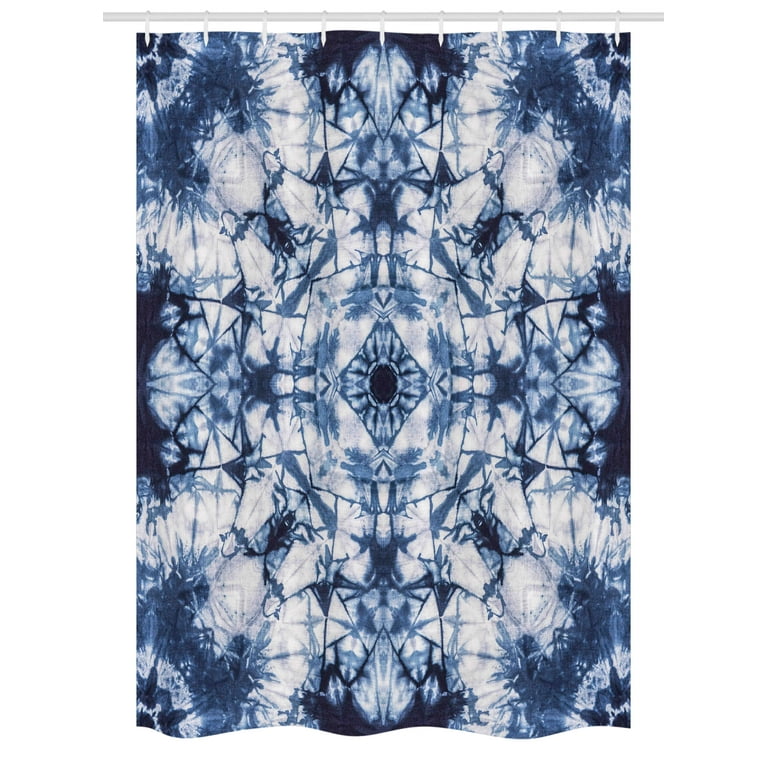The image features a shower curtain suspended from a white pole, held up by white rings. The shower curtain has a primarily white background with subtle gray undertones and is adorned with splatters of both dark and light blue hues, giving it a vibrant and artistic appearance. Dominating the center of the curtain is a diamond shape enclosing an oval, which is flanked by intricate, abstract designs that extend to the edges. These designs are varied in size and resemble spontaneous paint splatters, contributing to the curtain's modern and somewhat chaotic aesthetic. Notably, a faint, dark cross pattern lies subtly embedded in the overall design, adding to the curtain's futuristic and complex look.